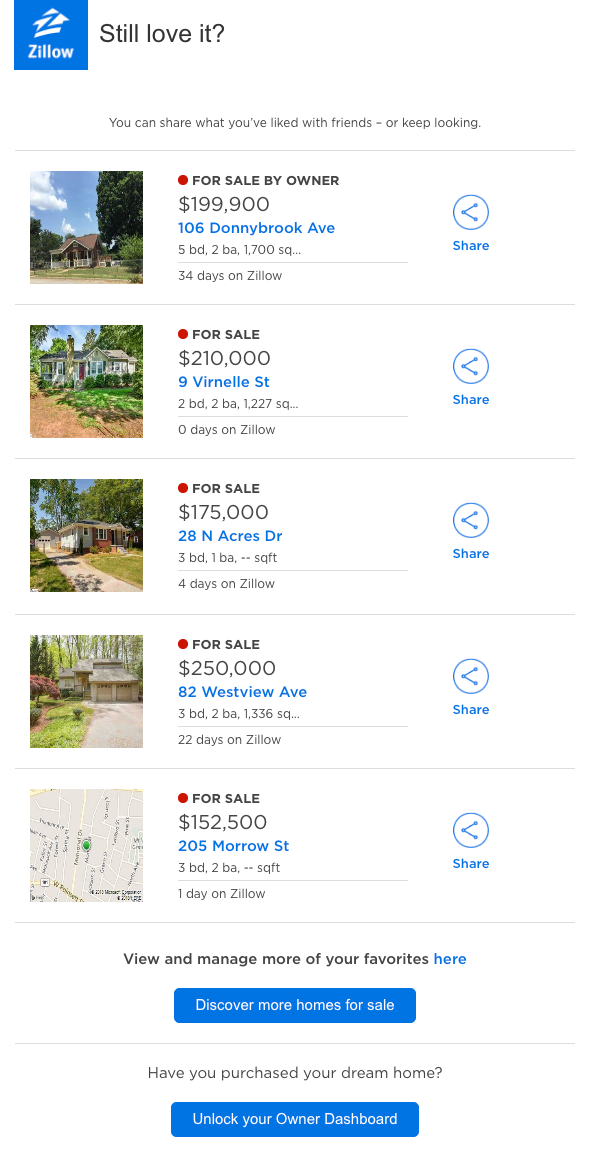The screenshot appears to be from the Zillow mobile app. In the top left corner, the familiar blue Zillow logo featuring a tilted house symbol with the word "Zillow" beneath it is clearly visible. Adjacent to the logo, "Still love it" is prominently displayed, followed by the message "You can share what you've liked with friends or keep looking." 

The main section of the image showcases five property listings. The first four listings feature images of houses, while the fifth listing only displays a map with a pinned location. The properties display various statuses, with four labeled “For Sale” and one at the top indicated as “For Sale by Owner.” Each listing includes a share button on the right-hand side, an address, and a price tag. Additionally, they all provide specific details such as the number of bedrooms, bathrooms, and total square footage. There is also a "Days on Zillow" counter showing how long each property has been listed: 34 days for the top property, 0 days for the second, 4 days for the third, 22 days for the fourth, and 1 day for the fifth.

Below the listings, the text "View and manage more of your favorites here" appears, followed by a hyperlink. Additionally, a blue button labeled "Discover More Homes for Sale" is prominently placed. Beneath this button, a question asks, "Have you purchased your dream home?" accompanied by another blue button labeled "Unlock Your Owner Dashboard."